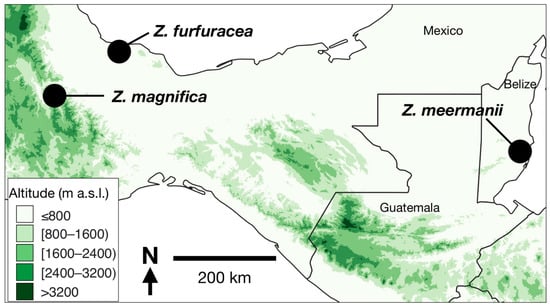This detailed map of Central America showcases the southern part of Mexico, most of Guatemala, and all of Belize. Additionally, small, unlabeled portions of two countries bordering Guatemala to the southwest are visible. The map features three marked locations with black circles, indicating specific species: Z. furfuracea and Z. magnifica in Mexico, and Z. mirmanii in Belize. The background is predominantly white, interspersed with various shades of green that depict altitude levels, as explained by the legend in the bottom left corner. This altitude legend ranges from below 800 meters (white) to above 3,200 meters (dark green) above sea level, with five specified intervals. A scale bar at the bottom signifies a distance of 200 kilometers, and an arrow marked 'N' points north, providing compass direction.